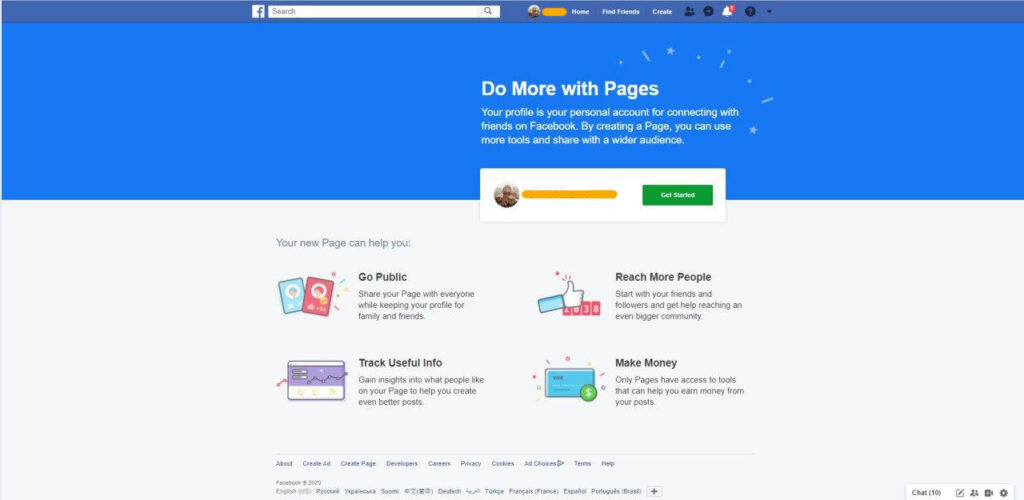The image depicts a Facebook interface encouraging users to create pages. The background is primarily blue with a prominent blue bar at the top. This bar hosts a white square containing a lowercase 'f' in blue, which is the Facebook logo, alongside a long white search bar.

Beneath the bar, white text reads, "Do more with Pages." A message explains, "Your profile is your personal account for connecting with friends on Facebook. By creating a page, you can use more tools and share it with a wider audience."

Further down, there's a small circular profile picture followed by a long yellow line, and next to it is a green rectangle with the text, "Get started."

The section below outlines options for creating a page:
- A blue and a red book icon labeled "Go Public."
- A thumbs-up icon labeled "Reach More People."
- A purple square labeled "Track Useful Info."
- A blue credit card icon with a green circle and a white dollar sign inside, labeled "Make Money."

At the bottom right corner, a gray word "Chat" is visible.

This detailed depiction provides a comprehensive overview of the Facebook page creation interface, highlighting essential visual and textual elements.